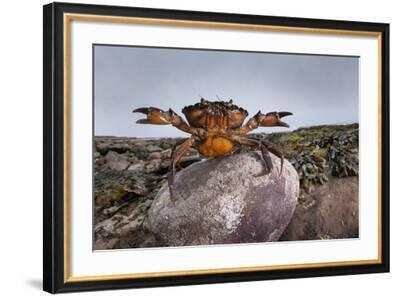The image features a detailed photograph encased in an ornate black and gold frame. The outer edge of the frame is black, encircling a gold etching. Inside this etching is a white, matte border that flatly secures the photograph. The photograph itself captures a dynamic scene of a brown and orange crab standing triumphantly on a large, rounded gray rock. The crab's claws are raised high, and it stands firmly on its long legs, suggesting a posture of alertness or display. Surrounding the crab are elements typical of a beach setting: patches of green seaweed, scattered rocks, and an expanse of sand. The backdrop is a sky painted in various shades of gray, indicating a cloudy or overcast weather condition, adding a moody atmosphere to the scene.